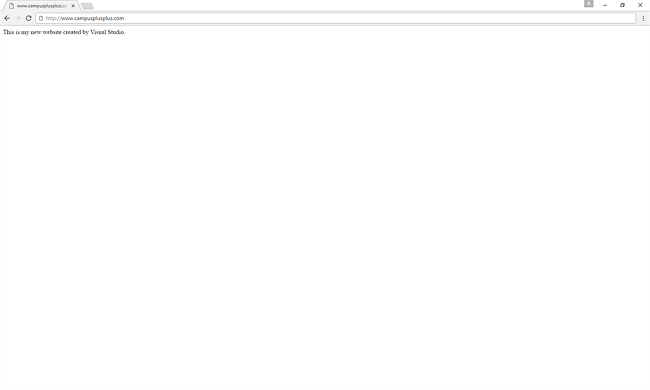A screenshot of a web browser window, which is predominantly white at the top, showcasing a very minimalist design. The browser appears to be either Chrome or a similar web browser, though the exact type is indiscernible. The URL in the address bar reads "www.campus++.com," albeit in extremely small text, roughly three pixels tall, making it difficult to read. The address bar extends across the width of the browser window. In the top right corner, the standard browser control buttons—close, minimize, and maximize—are clearly visible. Below the address bar, on the left side, there is a single line of text that starts with "This is my new..." followed by an unreadable word. The text ends with "created by Visual Studio," though the preceding word is too small to decipher. The rest of the browser window is blank and white, with no additional content.